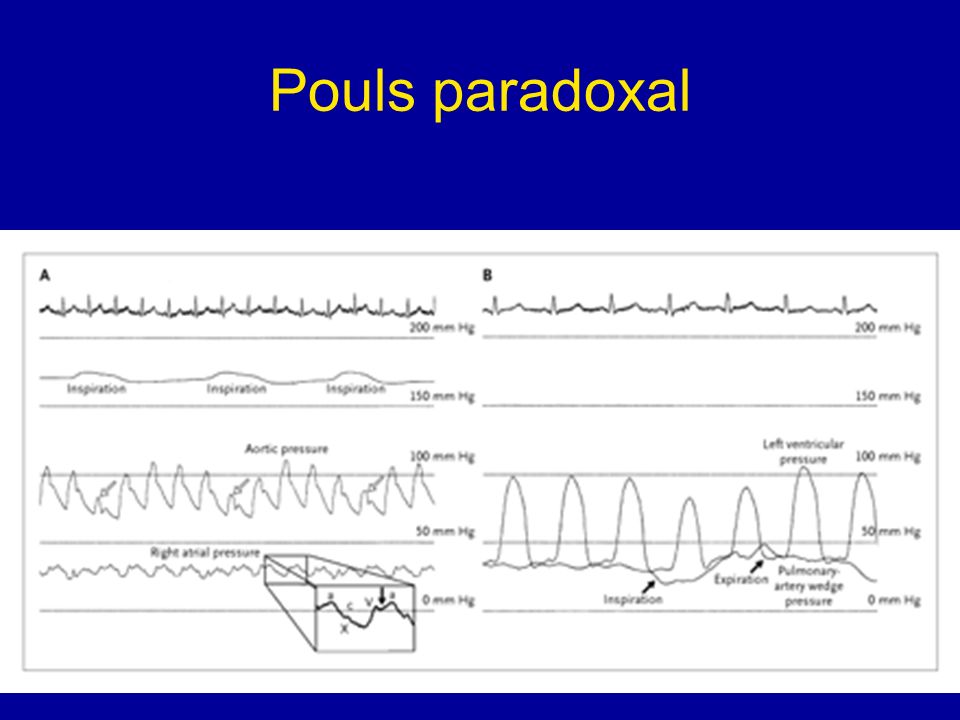The image is a PowerPoint slide displaying scientific graphs related to heart rate pulses, labeled "Pulse Paradoxal" at the top. The slide background is divided into three main sections: the top third is a deep blue rectangle featuring the text "PULSE PARADOXAL" in yellow, gold font. Below this header, there are two columns labeled A and B. Column A, located on the left, contains four graphs of various waveforms, while Column B on the right houses three similar waveforms. Both sets of graphs detail rhythms or measurements likely associated with electrocardiograms or different pulse waves, potentially indicating heart rate behaviors under certain conditions, such as arrhythmia or normal heartbeat fluctuations due to changes in blood pressure. The waveforms, depicted in black and white, range between 0 mm Hg and 200 mm Hg. Some of the lines on the graphs are marked with indistinct labels, possibly indicating pressures like aortic or left ventricular pressures, though the text is blurred and hard to read. At the very bottom of the slide is another small blue rectangle running across the width of the page.